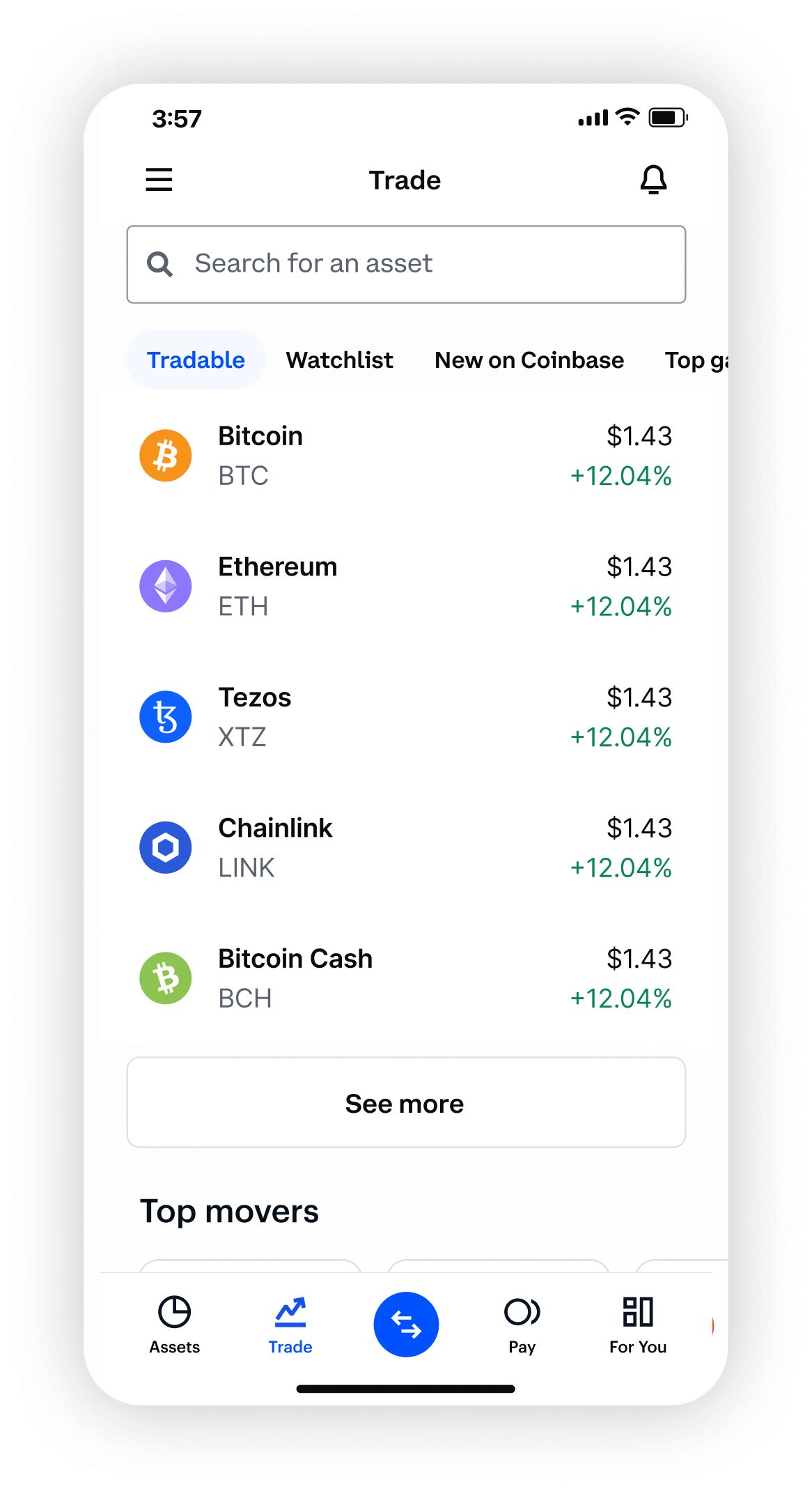A detailed and cleaned-up descriptive caption for the image:

"This image depicts a cryptocurrency trading application, most likely viewed on an iPhone due to the layout and design elements. The background of the app interface is white. The time displayed at the top of the screen is 3:57, with four Wi-Fi bars indicating full signal strength and the battery level at approximately 80%. 

At the top of the interface, on the left-hand side, there is a hamburger menu, and on the right, a bell icon. Between these icons, the title 'Trade' is prominently displayed. Below, there's a search bar labeled 'Search for an asset.' 

Further down, there is a slidable menu with several options. The first option on the left, highlighted in blue, is 'Tradable.' Other visible options, shown in black, are 'Watchlist,' 'New on Coinbase,' and 'Top GA...' with parts of other options like 'C-more' cut off.

The main content area lists various cryptocurrencies with dummy text for their values. At the top of the list is Bitcoin (BTC) with its distinctive white logo within an orange circle, valued at $1.43 (+12.04%). The subsequent cryptocurrency is Ethereum (ETH), indicated by a purple background behind its logo, also valued at $1.43 (+12.04%). This pattern continues for Tezos (XTZ) with a unique logo, Chainlink (LINK) with a hexagonal logo, and Bitcoin Cash (BCH), all displaying the same dummy text ($1.43, +12.04%).

At the bottom of the interface, there are navigational buttons labeled 'Assets,' 'Trade,' 'Forward,' 'Backward,' 'Pay,' and 'For You,' facilitating easy access to different sections of the app."